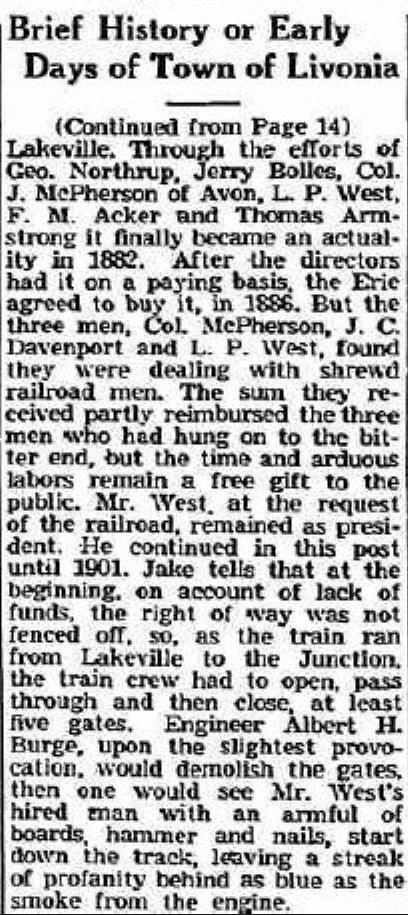This newspaper clipping, a low-quality JPEG scan, provides a detailed continuation of the article "Brief History or Early Days of Town of Livonia" from page 14. The article recounts the establishment and struggles of the town of Livonia, particularly Lakeville, through the efforts of key figures like George Northup, Jerry Bowles, Colonel J. McPherson of Avon, L.P. West, F.M. Acker, and Thomas Armstrong. The text, compressed and somewhat difficult to read, narrates how the town finally became a reality in 1882 once the directors had made it financially viable. The Erie Railroad agreed to purchase it in 1886, although the deal proved challenging due to shrewd negotiations by railroad men. Despite some reimbursement, the three main contributors, including Colonel McPherson, J.C. Davenport, and L.P. West, were not fully compensated for their time and efforts. Mr. West continued as president at the railroad's request until 1901. The column vividly describes how, due to the lack of fencing along the right of way, train crews frequently dealt with the inconvenience of operating gates. Engineer Albert H. Burge, known for his temper, would sometimes demolish these gates, leaving Mr. West's hired man to repair them amid a trail of colorful language, as thick as the engine's smoke.